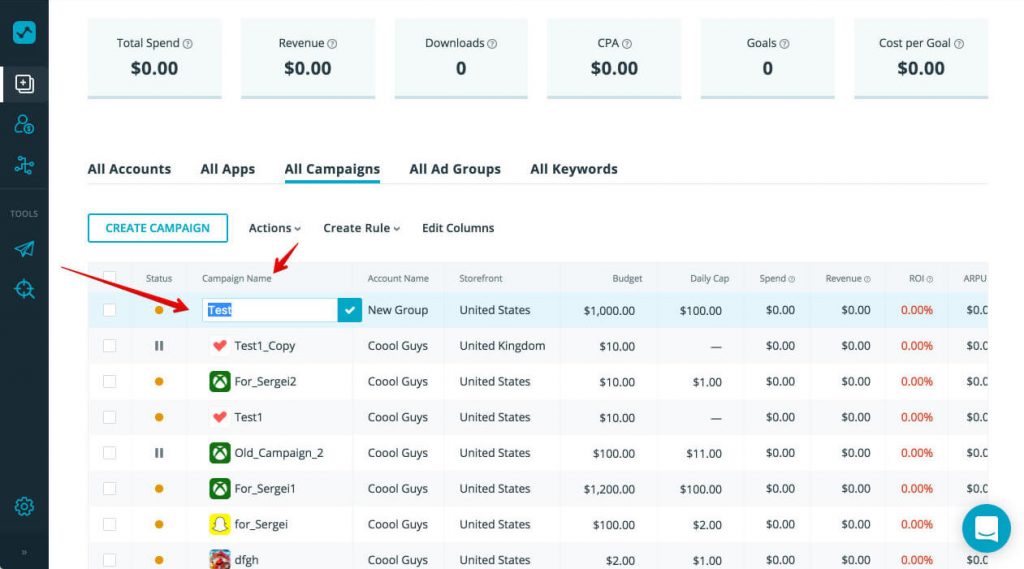The image shows a detailed dashboard interface of an advertising management platform. At the top, there are six gray rectangular boxes displaying the following metrics from left to right: Total Spend ($0), Revenue ($0), Downloads (0), CPA ($0), Goal (0), and Cost per Goal ($0). Below these metrics, a navigation menu with the items “All accounts”, “All apps”, “All campaigns”, “All ad groups”, and “All keywords” is present, with the “All campaigns” option underlined in light blue.

Further down, there are options for managing campaigns, including “Create Campaign”, “Action”, “Create Rules”, and “Edit Columns”, with “Create Campaign” emphasized in blue capital letters and enclosed within a blue rectangular outline. 

Beneath these options, a spreadsheet-like table features several columns with headers and data entries. A red arrow points to the “Campaign Name” column header. Another red arrow points to a text box labeled “Test”, which also contains a blue square with a white checkmark on the right side. Below this, the data entries in the table include “test1_copy”, “4_surgery_2”, “test1”, and “old_campaign_2”.